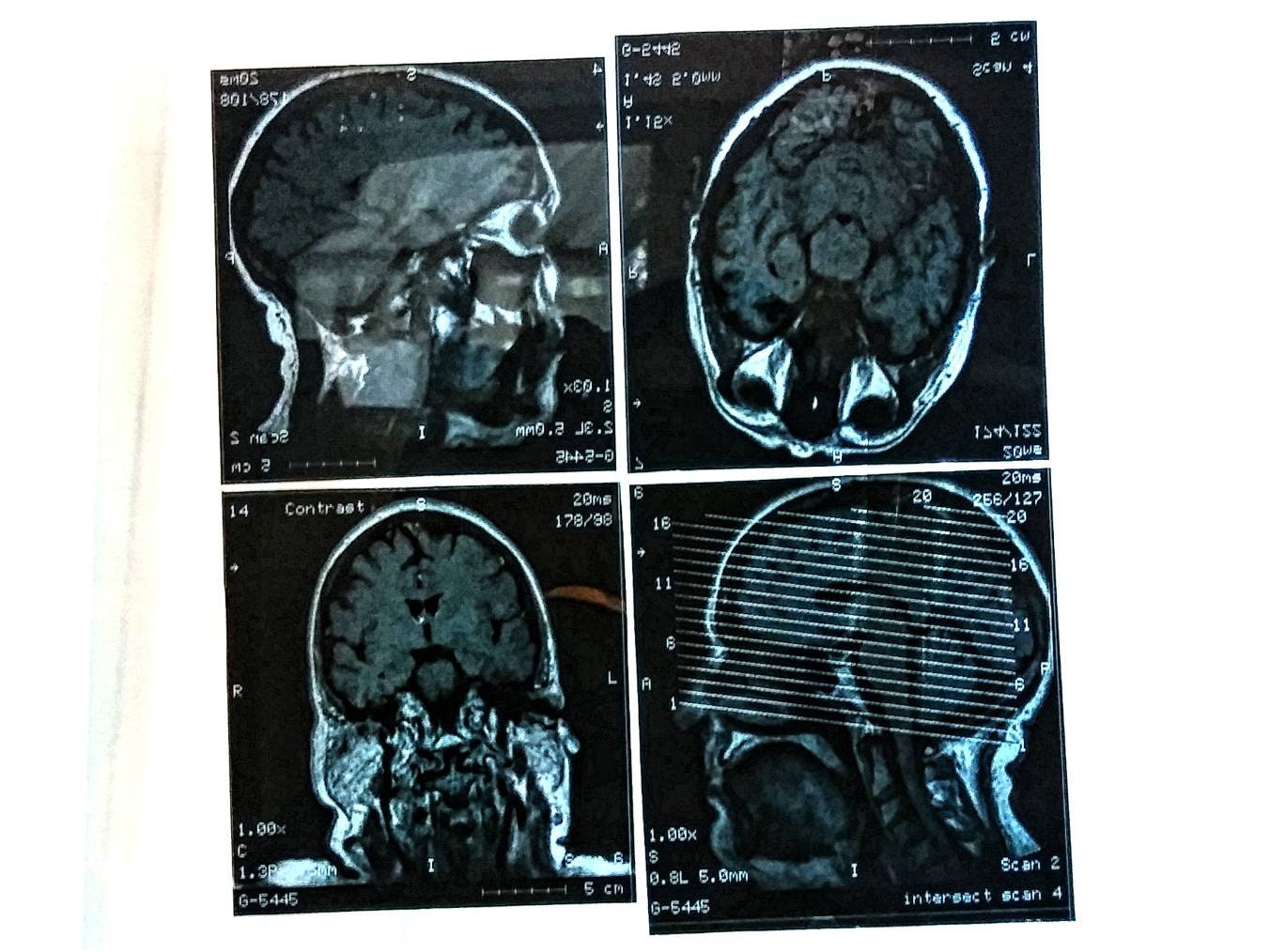This scientific photograph displays a series of four detailed medical scans of a human skull and brain, arranged in a 2x2 grid fashion. 

- **Top Left Image**: A side profile x-ray showcasing the skull's outline, brain, and eye cavities. The background is predominantly black, with white and gray tones denoting the anatomical structures.

- **Top Right Image**: Another x-ray view from above, illustrating the top view of the skull, brain, and eyeballs. This image also features a black backdrop with the prominent white-gray contrast of the skull.

- **Bottom Left Image**: A posterior x-ray view, highlighting the back of the skull and brain. This view provides more details of the brain's structures and the cavities leading into the neck.

- **Bottom Right Image**: A cross-sectional x-ray of the left-hand side of the skull, revealing the detailed anatomy of the cheek, brain, and the base of the skull. This scan includes annotations, numbers, and coordinates, possibly indicating specific areas of interest for the scan.

All images possess a color scheme dominated by black, white, and some shades of blue-gray, with various annotations and measurement markers present, particularly in the bottom right scan.